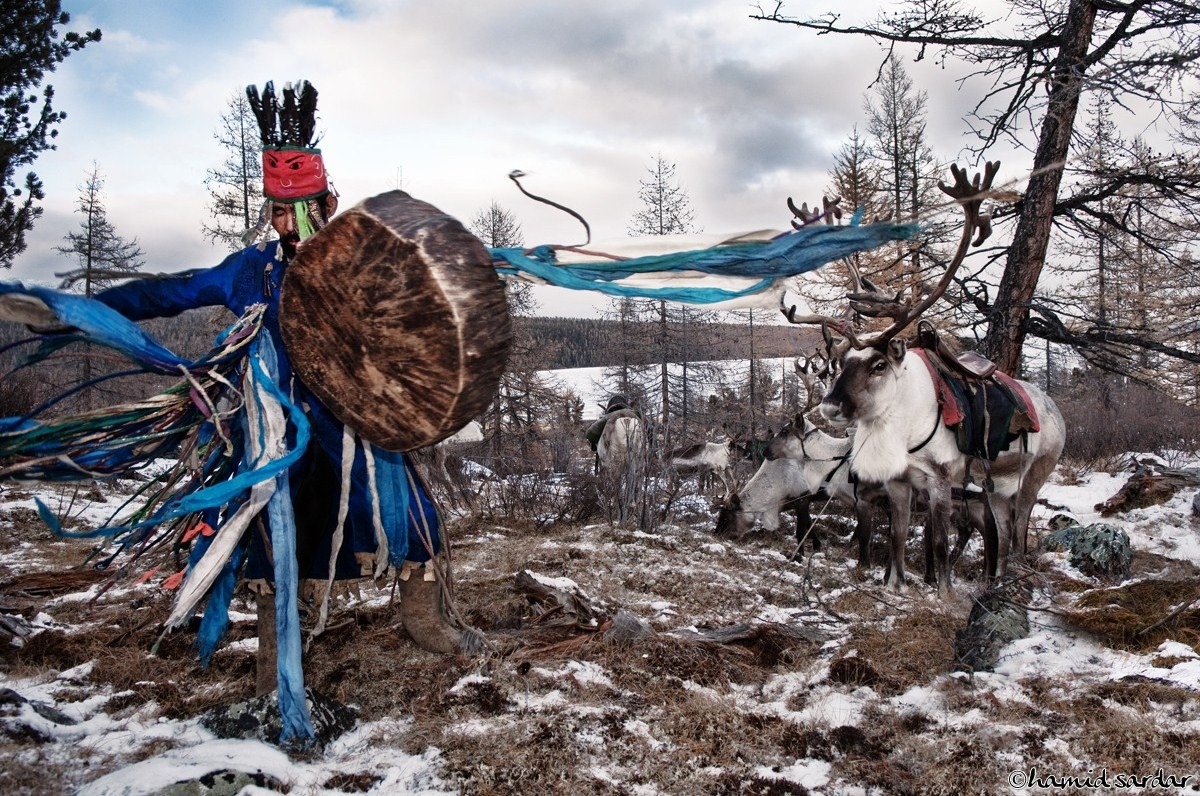In this color photograph set in a woodland forest during wintertime, an indigenous man adorned in traditional attire stands among the barren, brown trees, with patches of snow blanketing the ground. The man, positioned to the left side of the landscape-oriented image, wears a striking blue long-sleeve top, sharply contrasting with the muted tones of the forest. His outfit features strands of fabric in blue and white, which cascade around him, adding a dynamic movement as if he is mid-dance or preparing to strike the giant wooden drum or trunk before him. His red tubular headdress, adorned with black feathers that protrude from the top, further emphasizes his vibrant presence. Partially obscured by fabric strands, his face is oriented downward, yet he remains an enigmatic focal point of the photograph.

To his right, a horizontal overhead rope draped with blue and white scarves extends across the scene. Beneath this, two reindeer with long antlers and white coats, marked by black faces, stand in profile, gazing into the viewer's eyes while one grazes in the background. The reindeer are outfitted with saddles and saddlebags, adding to the intricate details of the image. The background features a dense array of leafless trees under a sky filled with ominous dark gray clouds, enhancing the eerie and surreal atmosphere of the photograph. The overall style is that of photographic representationalism realism, giving it an almost surreal yet highly detailed depiction of the elements contained within. An illegible credit resides in the bottom right corner, completing the image's detailed description.